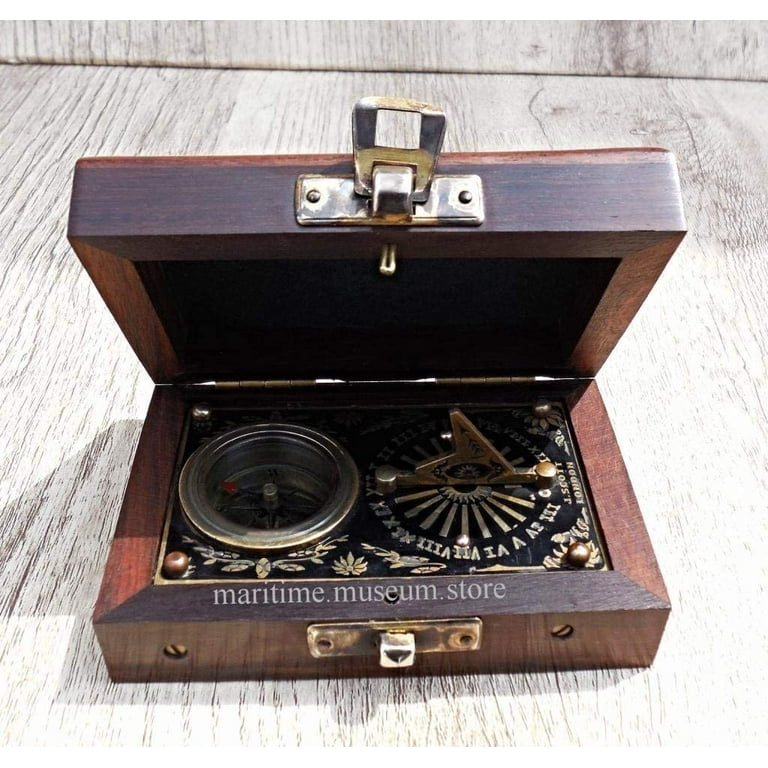A beautifully crafted, antique-looking sextant sits in an exquisitely made wooden box. The box, dark brown with lighter brown accents, is positioned on a bleached, white wooden surface, possibly a bench by the sea and illuminated by sunlight. The lid of the box, held open by a brass clasp, reveals the words "Maritime Museum Store" inscribed inside. Inside the box, the sextant features two primary circular components – on the left, a compass displaying directional information, and on the right, a clock-like dial with Roman numerals and golden hands. Between these circles are intricate, flower-like designs, and there's a notable golden piece protruding, indicating the sophisticated craftsmanship. The overall scene captures a sense of nautical history and meticulous artisan work against the rustic backdrop and natural lighting of the outdoors.